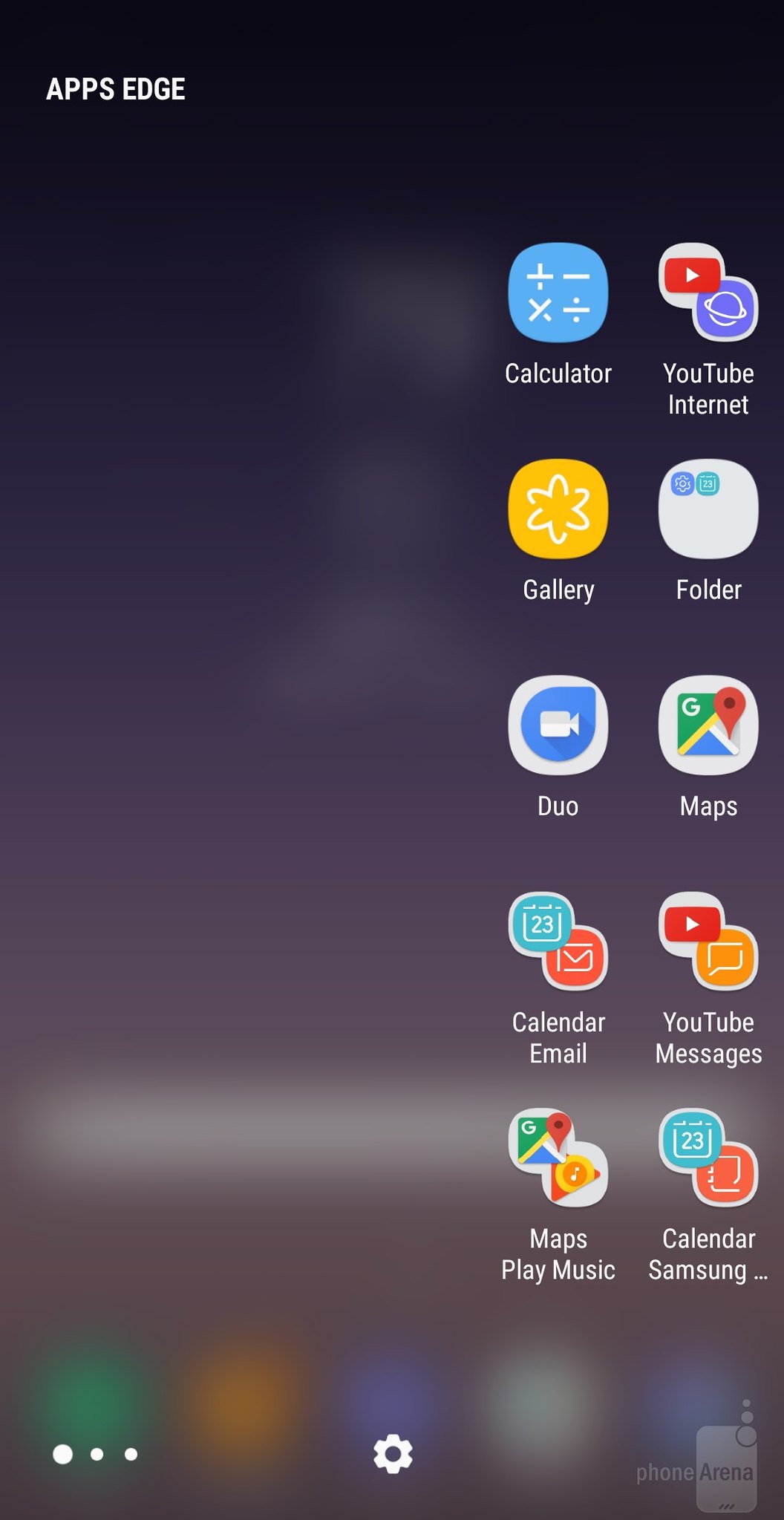The image is a screenshot of a cell phone screen, specifically focusing on the "Apps Edge" feature commonly found on Android devices. The screen shows a prominent black bar at the top with the label "Apps Edge" displayed in white text. The majority of the screen is covered by an opaque overlay, through which the underlying full screen is partially visible, indicating that the overlay is a pop-out edge bar.

On the right-hand side of this overlay, there are ten app icons arranged vertically. The apps are listed as follows:

1. **Calculator**, **YouTube**, and **Internet** - grouped closely together.
2. **Gallery**
3. A folder containing two unidentified apps that are too small to discern.
4. **Duo**
5. **Maps**
6. **Calendar** and **Email** - grouped together.
7. **YouTube** and **Messages** - grouped together.
8. **Maps** and (presumably) **Play Music** - grouped together.
9. **Calendar** and (presumably) **Samsung** app - grouped together.

This organization suggests a personalized selection of frequently used applications accessible from the edge bar.

At the bottom of this opaque area, there are three navigation elements:
- Three dots located in the bottom left corner.
- A settings icon situated in the center.
- A logo or watermark on the bottom right, which seems to read "PhoneArena." The word "Phone" is in gray, while "Arena" is in black on a gray background.

The presence of app icons and specific UI elements indicates this is an Android phone. The screenshot reveals other background apps, confirming that this is a pop-out edge bar feature used for quick access to selected applications.